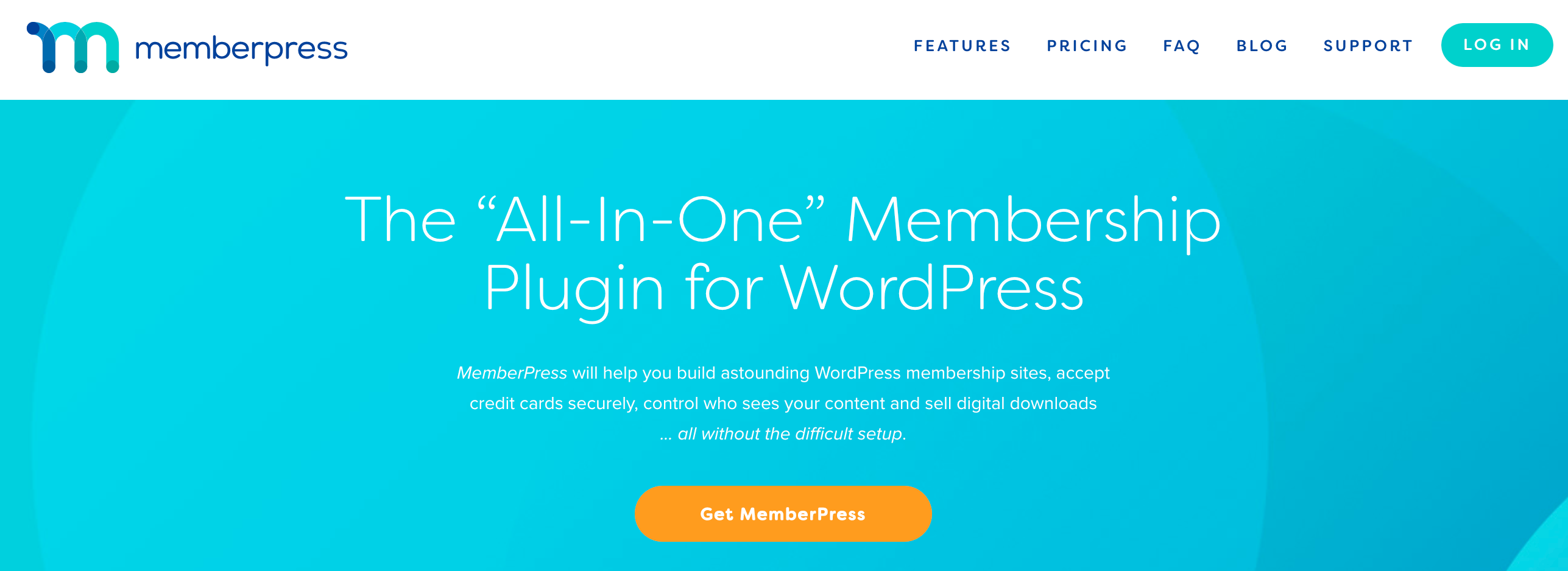A detailed caption for the screenshot would be:

"This desktop screenshot captures the homepage of MemberPress, a comprehensive membership plugin for WordPress. At the top of the screen, the MemberPress logo is displayed next to the name 'MemberPress,' accompanied by a navigation menu with options such as Features, Pricing, Frequently Asked Questions, Blog, Support, and a Login button. Central to the page, an advertisement describes MemberPress as the 'all-in-one membership plugin for WordPress,' boasting capabilities to help build impressive membership sites, securely process credit card transactions, control content access, and sell digital downloads—all without complex setup. Highlighting the page's call to action, a large orange button at the bottom center reads 'Get MemberPress,' inviting users to proceed with purchasing the plugin. The color scheme primarily features light blue backgrounds with white text, creating a clean and professional look."